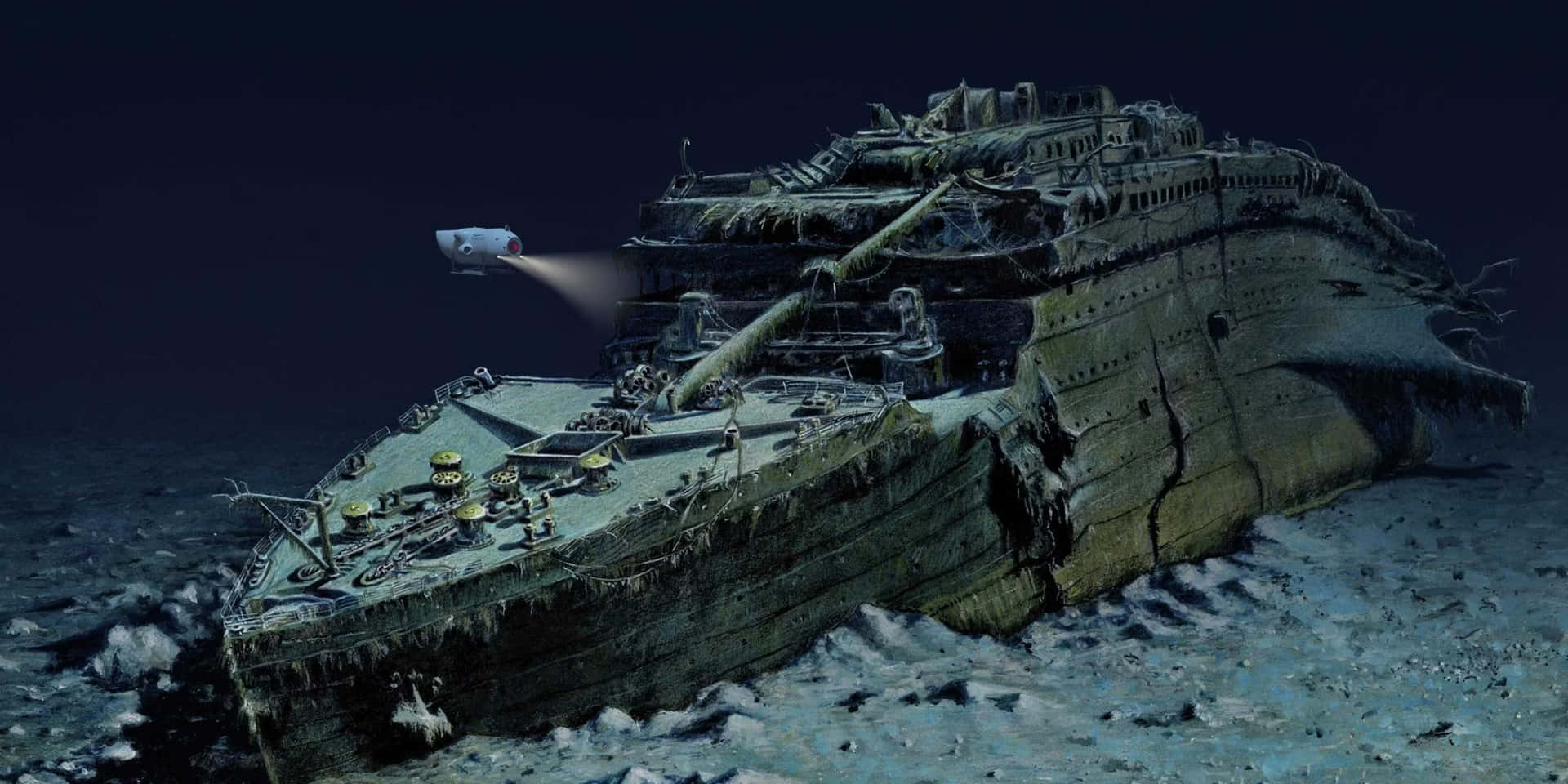This detailed, artistically rendered underwater scene depicts a rusted shipwreck, possibly representing the Titanic or another substantial maritime disaster, lying eerily on the ocean floor amidst piles of sand. The ship, encrusted with green moss and showing signs of structural collapse, extends diagonally from the bottom left to the upper right of the image. In the top left corner, a sleek, modern-looking submersible vehicle shines its lights onto the wreckage, suggesting an active exploration or research endeavor. The clarity of the water, with no visible marine life, enhances the eerie atmosphere of the scene. While the image displays an incredible level of detail, suggesting an artist's recreation rather than a genuine photograph, it still provides a hauntingly realistic glimpse of what it might look like at the depths where the Titanic or a similar shipwreck lies.